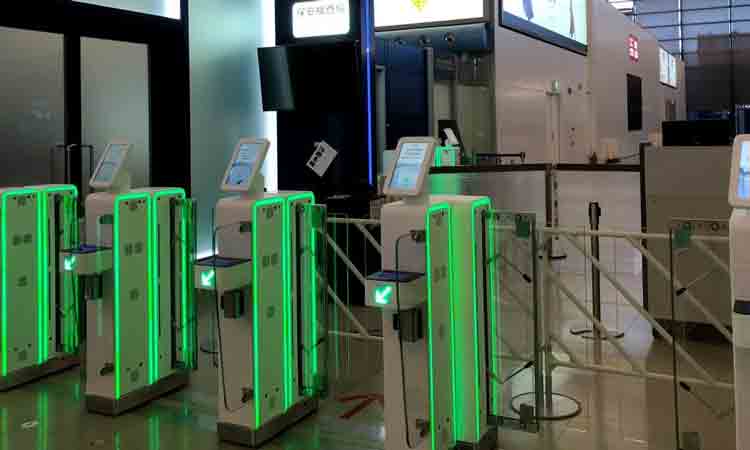This horizontally aligned rectangular photograph captures a high-security entrance area inside a modern building, reminiscent of an airport security checkpoint. The scene showcases four sleek, white security gates arranged from left to right. Each gate is integrated with green LED accents, including a prominently displayed green arrow pointing diagonally left, directing passage when the gates are open. However, all gates are currently closed, secured by metal barriers. Each station is equipped with a digital screen or tablet on top and a small box below, possibly for hand scanning or access control. The background reveals an expansive walkway with a doorway to the left and illuminated signs adorned with black symbols, suggesting a non-American location. The flooring consists of tan-colored tiles, contributing to the overall modern and secure atmosphere of the setting.